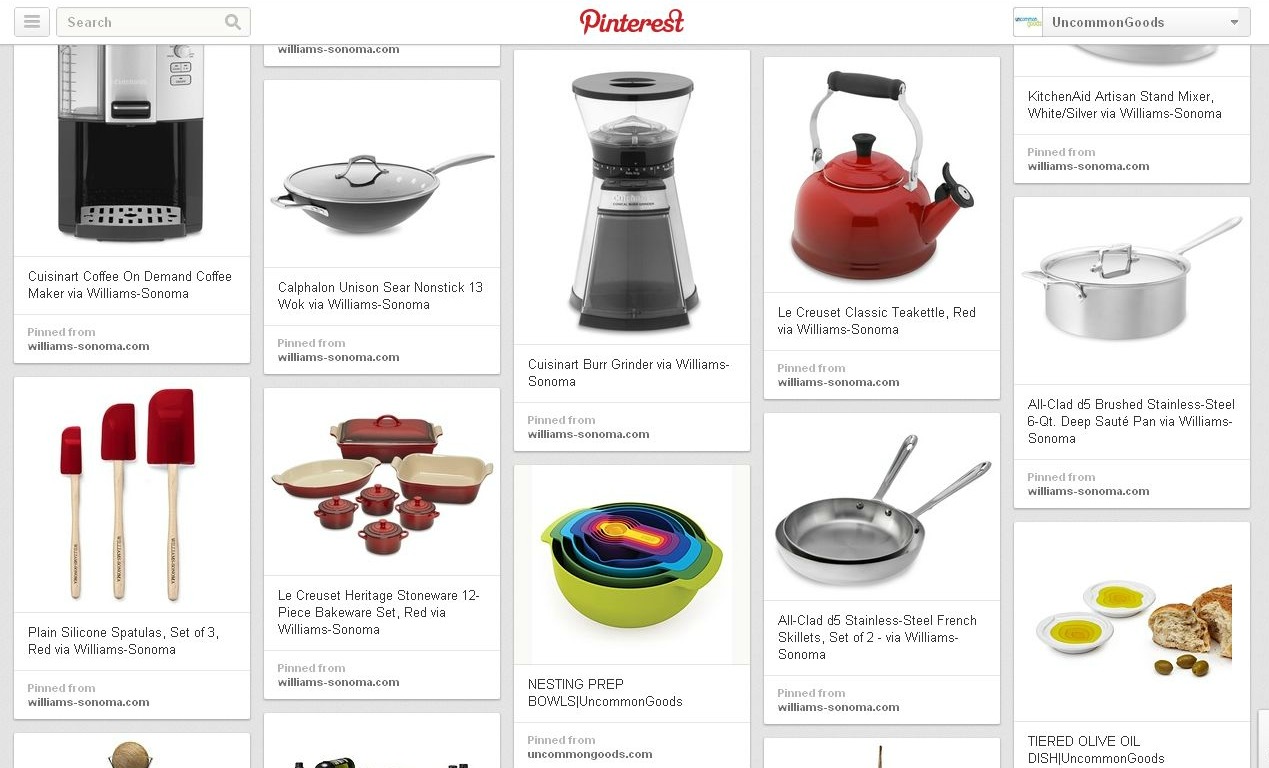This screenshot from Pinterest showcases the platform's interface, prominently featuring the Pinterest logo at the top of the page. On the left side, there's a search box, while the right side displays a dropdown menu labeled "Uncommon Goods." The main section of the screen is filled with various kitchen and household items, including an image of the Cuisinart Coffee on Demand coffee maker. Several other Cuisinart products, along with a grinder and a Calphalon pot, are also visible. Each item has a brief typed description in black lettering, although the text appears somewhat faded and difficult to read. The images, however, are clear and vibrant. Notable items include a set of nesting bowls in varying shades of green, a collection of red Le Creuset bakeware, and several olive oil trays.